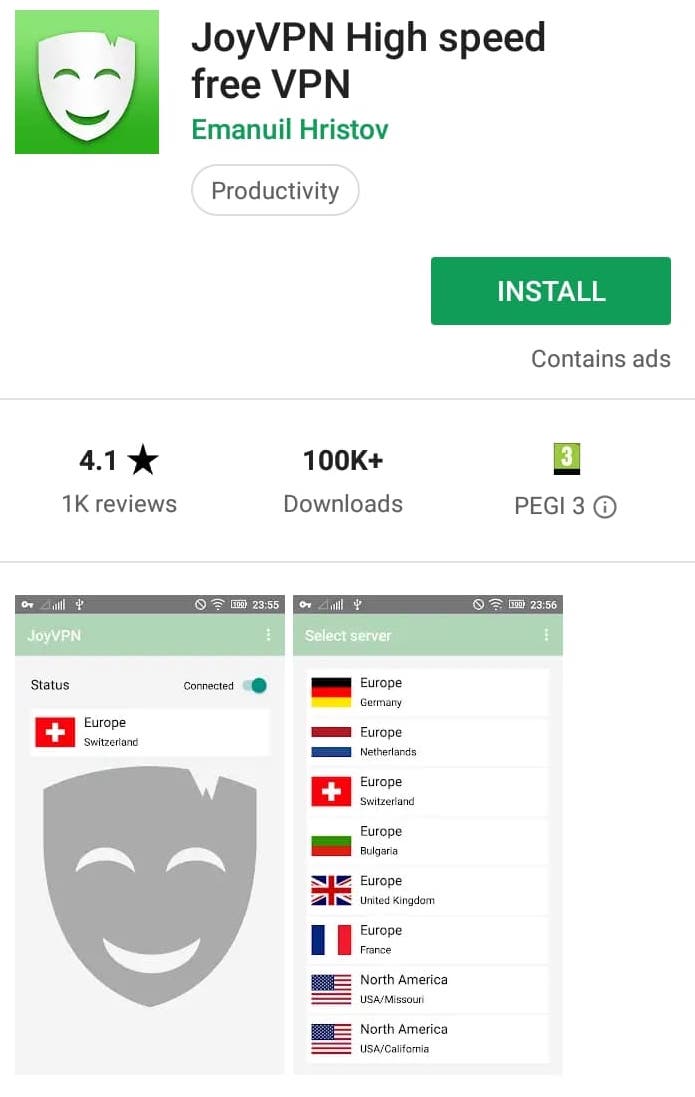**App Store Screenshot Description: Joy VPN**

The image appears to be a detailed screenshot from a phone displaying the Play Store page for an application called "Joy VPN High Speed."

- **Background and Layout**: The entire page is set against a clean, white backdrop. There are no typical phone icons at the top, providing an uninterrupted view of the app information.
  
- **Logo and App Name**: On the upper left-hand corner, there is a green square containing a distinctive white mask icon. The mask features a smiling face, with crescent moon-shaped eyes tilting upwards and a crescent-shaped smile. There is a small chip-like detail on the mask's head.
  
- **App Title and Developer**: To the right of the green logo box, the title "Joy VPN High Speed" is displayed in bold black text. Directly beneath it, "Free VPN" is written, followed by the developer's name, "Emanuil Hristov," in green font.

- **Category and Installation**: Below this, a white bar outlined in gray categorizes the app under "Productivity," and next to it on the right, a prominent green bar labeled "Install" allows the user to download the app. Under the install button, "Contains Ads" is indicated in black text.

- **App Rating and Downloads**: A thin gray line separates the install section from the app rating details. Below the line, the app is rated "4.1" stars, shown next to a star icon. "1K Reviews" is noted adjacent to the rating, followed by "100K+" symbolizing the number of downloads. Additionally, a green box with a white number "3" inside denotes the app’s PEGI 3 rating, suitable for all age groups. There is also a white circle outlined in gray containing a lowercase 'i,' likely an information icon. 

- **Screenshots Provided**: The lower part of the image features two app screenshots, side by side:
  - **Left Screenshot**: Displays the main interface of Joy VPN. The top bar includes typical phone symbols such as service strength, Wi-Fi, and battery life, presented in a compact format with a timestamp. The interface shows "Joy VPN" in white at the top, followed by an icon with three vertical dots. The text "Status" and "Connected" indicates a successful connection. A bar beneath shows a green circle on the right. Further down, a selection with a red box containing a white plus symbol (resembling the Swiss flag) points to "Europe - Switzerland." The gray logo of the mask is also visible, signifying the app's branding.
  
  - **Right Screenshot**: Also features the main interface but highlights the server selection process. Under "Select Server," a list of locations is shown with corresponding flags and country names. The regions are organized by continents:
    - Europe: Germany, Netherlands, Switzerland, Bulgaria, United Kingdom, France.
    - North America: USA (Missouri, California).

This detailed description captures the intricacies of the screenshot, providing an informative and thorough overview of the "Joy VPN High Speed" app page from the Play Store.